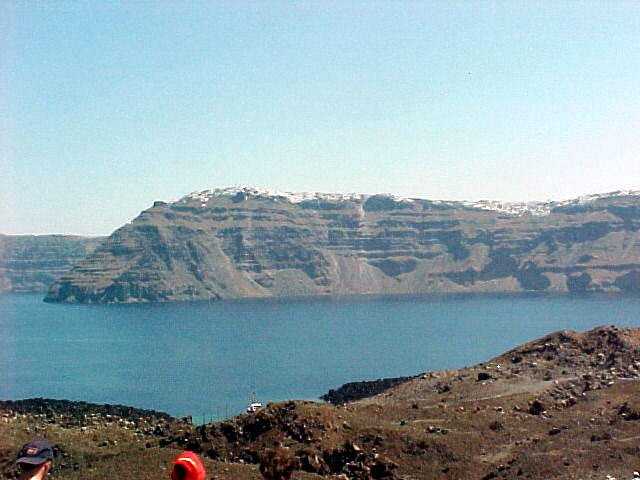This photograph captures a breathtaking panoramic view of a large mountain range and an expansive lake under a clear, light blue daytime sky. The serene lake in the center of the image mirrors the blue sky, creating a mesmerizing effect. Majestic mountains embrace the lake, with their peaks adorned with patches of snow, indicating a higher altitude. In the foreground, the photograph reveals a plateau, suggesting that the photographer is positioned on a similar elevated terrain, giving the image a grand and encompassing perspective.

Amid the rugged beauty, two hikers are visible in the bottom left corner; one is wearing a blue cap, and the other an orange hoodie, adding a sense of scale and human presence to the vast landscape. The scene is reminiscent of the grandeur of the Grand Canyon but with distinct mountainous features and a placid body of water. The overall atmosphere is calm and picturesque, capturing the essence of untouched natural beauty.